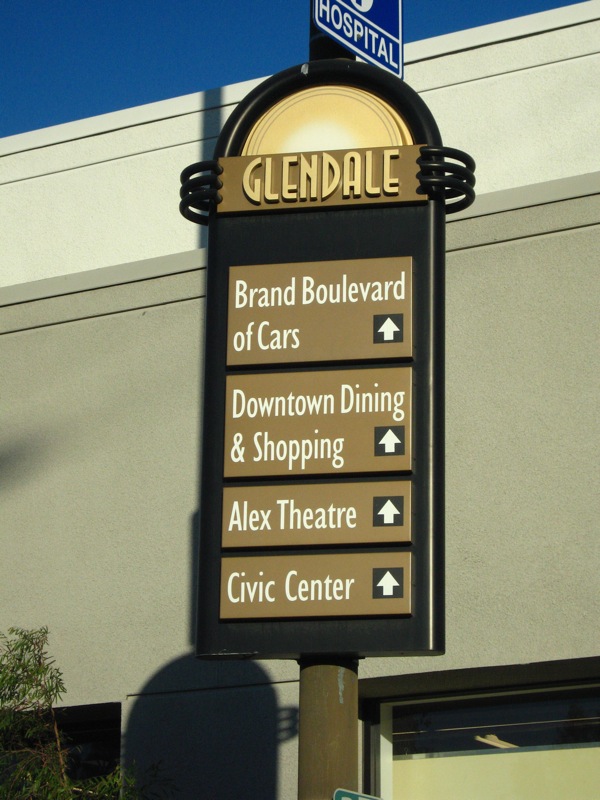The image depicts a first-person perspective of signage attached to a steel pole at an outdoor mall. The top of the sign is arched and colored yellow, resembling a rising sun. Below the arch, the word "Glendale" is prominently displayed in light yellow against a brownish-green background. The main part of the sign has four rectangular sections, each with white text on a brown background and a white arrow pointing up. The sections read from top to bottom: "Brand Boulevard of Cars," "Downtown Dining and Shopping," "Alex Theatre," and "Civic Center." Above this main sign, there is a smaller blue sign with the word "Hospital" in white letters. The entire sign is bordered in black, and the pole supporting it is visible at the bottom of the image. In the background, part of a building and a clear sky transitioning from blue and white at the top to gray in the middle can be seen, along with some windows and a shadowed object.